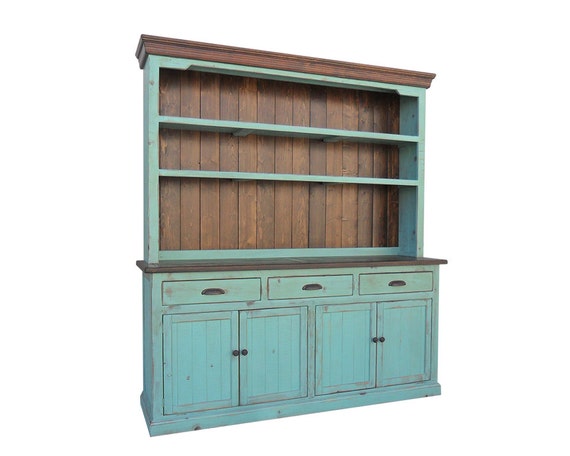The image captures a bright and naturally lit scene featuring a vintage, farmhouse-style hutch set against a white-walled backdrop, likely in a dining room or kitchen. The hutch is primarily painted in a soothing robin's egg green, reminiscent of mint or teal, with natural wood accents that include a dark brown, possibly mahogany, countertop and matching drawer handles. The piece is designed for both functionality and display, featuring three empty wooden shelves on the top for showcasing China or dishes. The lower section comprises a flat surface perfect for serving during gatherings and three individual pull-out drawers, followed by two double-door cabinets for additional storage. The meticulous attention to detail and the rustic charm make this furniture piece a versatile and elegant addition to the room.